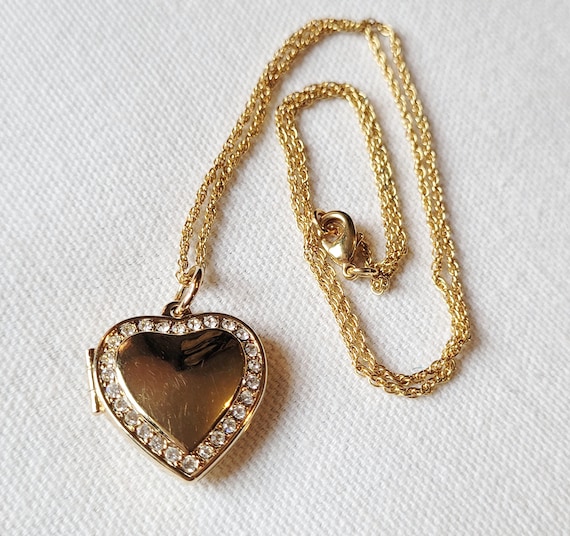This detailed image features a gold heart-shaped locket adorned with rhinestones set against a white fabric background. The locket, likely made of costume jewelry, has a hinge on its left side, suggesting it can be opened to reveal a space inside. The locket is encased in a heart-shaped golden frame with rhinestones running around its entire edge, giving it a sparkly, elegant appearance. At the top of the heart is a small hole where the locket attaches to a golden chain, which is neatly looped and curled to prevent tangling. The reflective surface of the locket captures the ambient light, giving it a shiny, well-loved look. The delicate golden chain, featuring a lobster claw clasp, loops elegantly over itself. The pristine white background enhances the gold's glow, making the locket the image's centerpiece.